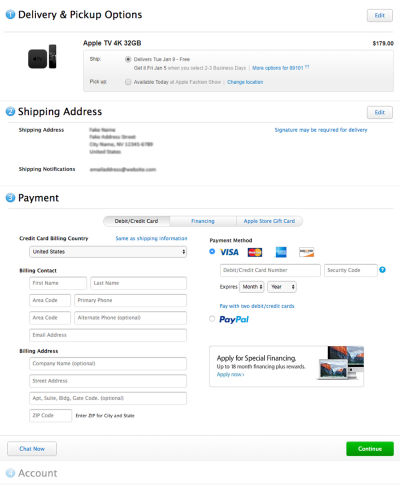The image depicts a vertically rectangular screen grab from a retail website, most likely the Apple Store. The top-left corner displays the options for delivery and pickup, while an 'Edit' button is located at the top-right corner. Below this, the product listed is the Apple TV 4K with 32GB storage, priced at $179. There are options for choosing between different delivery or pickup methods, but these are blurred and unreadable.

Further down, the "Shipping Address" section is seen, featuring fields for entering the shipping address and opting for shipping notifications. Below this is the payment area, showcasing three side-by-side buttons in the center for Debit/Credit Card, Financing, and Apple Store Gift Card. 

Additional fields are available for entering credit card details, billing contact information, and billing address, with a PayPal option also provided. Towards the bottom, there is a 'Chat Now' button on the left and a green 'Continue' button on the right.